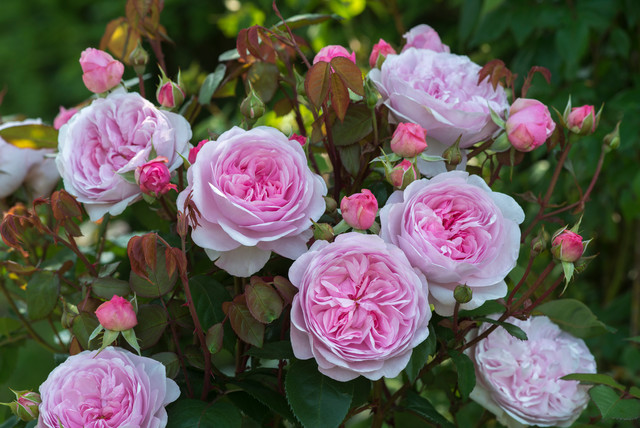This is a beautifully detailed and close-up photograph of a healthy bush of double roses. The flowers, in a light baby pink or ballerina pink shade, are exquisitely clear and vivid, with about six or seven fully bloomed roses showcasing darker petals in their centers and lighter petals surrounding them. The image also captures numerous buds, totaling around 13 to 14, that have yet to open. The leaves are a lush, dark green, with some appearing reddish, and some have a spiky texture, indicative of thorns. In the foreground, the focus is sharp, highlighting the intricate lines and details of the rose petals and the texture of the leaves, including a distinct spiky one under one of the fully bloomed flowers. The background consists of more greenery, softly blurred to emphasize the bush in front. The scene is partially sunlit, suggesting it is either mid-morning or early afternoon, adding a natural brightness to the vibrant colors of the roses and casting subtle shadows in the background. The overall impression is one of a vibrant and beautifully composed natural bouquet.